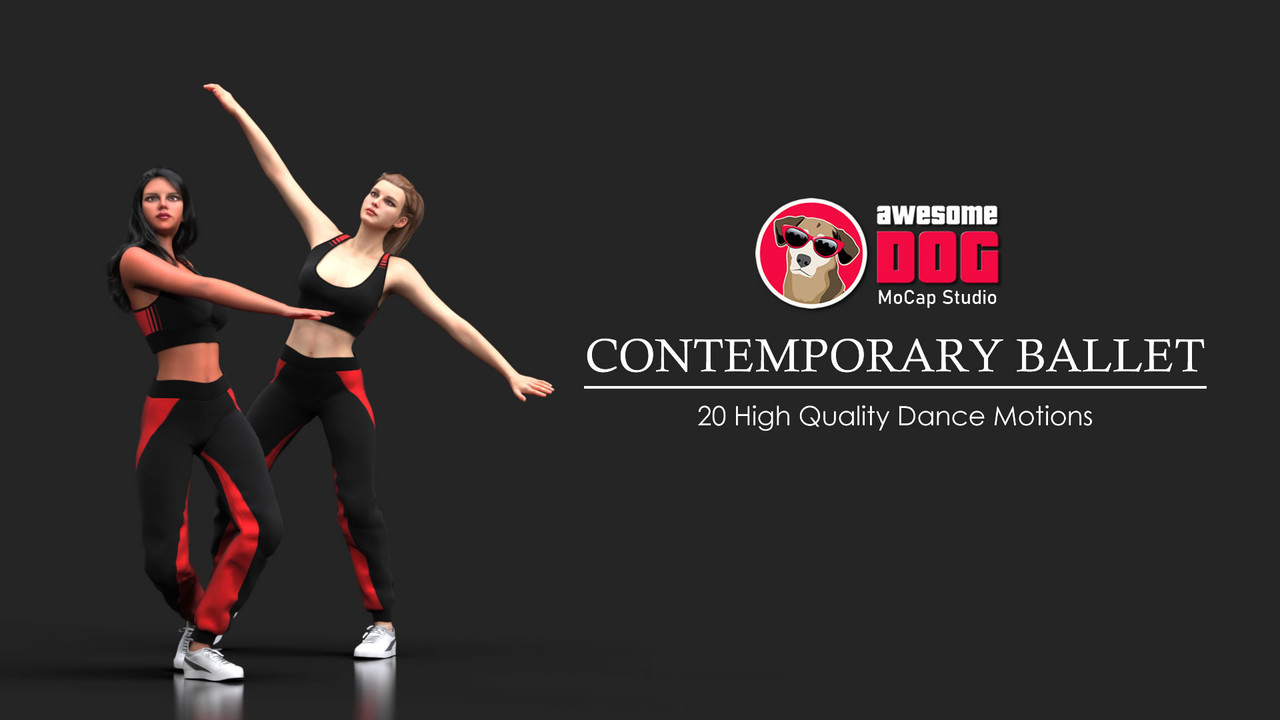The advertisement features a sleek dark gray, almost black, background. Dominating the left side are two 3D-rendered female dancers, dressed in matching sports attire that includes black tank tops with red accents and black sweatpants featuring red detailing on the legs. Both dancers are wearing white Puma sneakers and are in mid-dance pose with their arms outstretched. The dancer on the right has peach-white colored skin and brown hair, while the dancer on the left has a darker skin tone and darker brown hair.

On the right side of the graphic, there is a small circular logo with a brown dog wearing red sunglasses, outlined in white. Adjacent to this logo is bold text that reads, "Awesome Dog," with "Awesome" in white and "Dog" in large red letters with a black outline. Below this, in a different font and underlined, the text reads "Contemporary Ballet." Further down, it states, "20 high-quality dance motions" in white text, presenting the offering of the mocap studio.